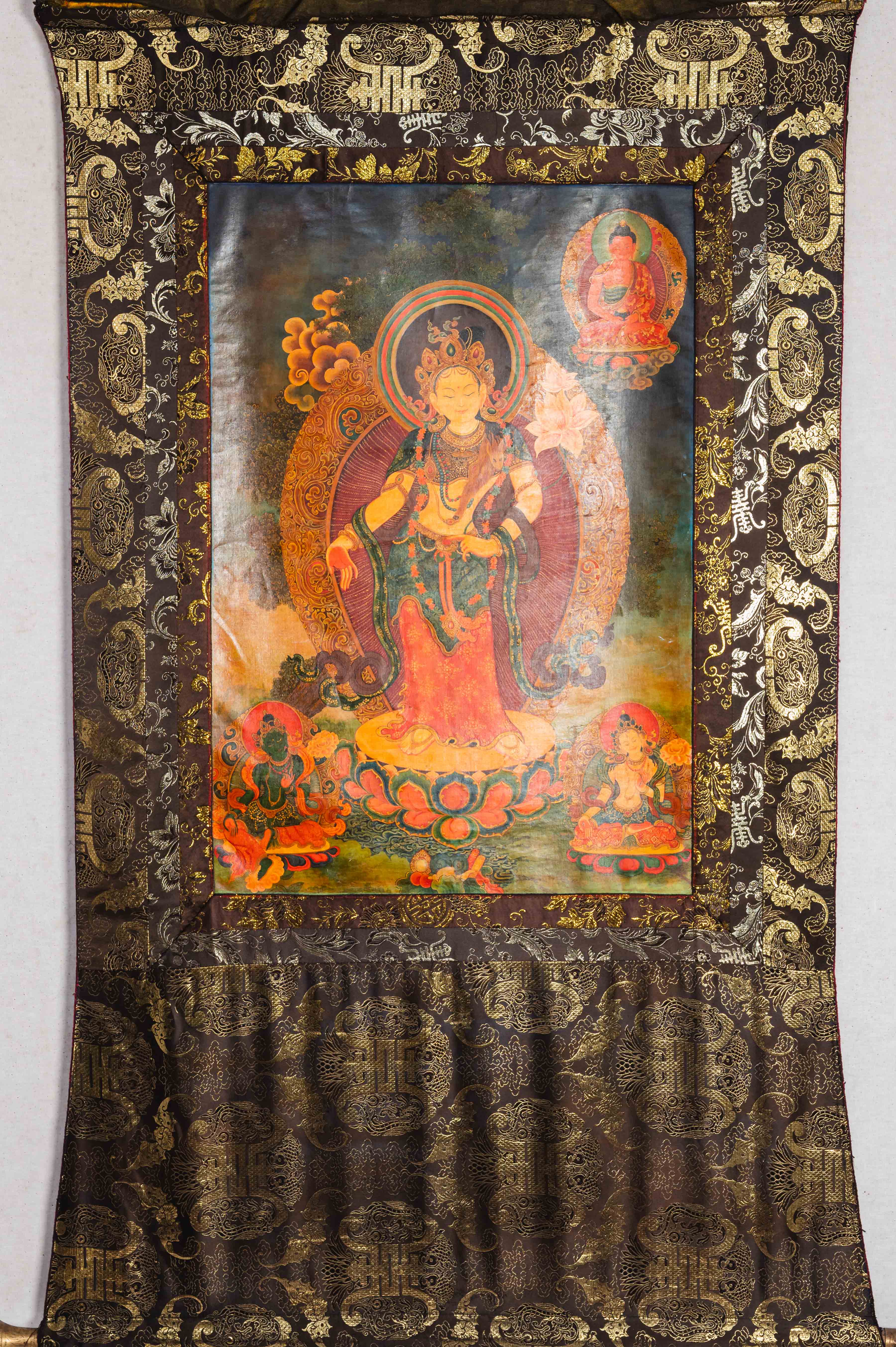The image features a highly detailed cultural tapestry hanging on a white wall. The tapestry rests on a brown, gold, and silver scarf with intricate gold trims and leaves, and a white surface is visible beneath the scarf. At the center of the tapestry, an ornate illustration depicts an Asian goddess adorned in a luxurious reddish-orange and green dress. She wears a gold crown and is encircled by a green and yellow snake. Behind her is a colorful background bearing the same hues as her attire. Surrounding her are multiple deities, including a meditative Buddha with a matching background in the upper right, and two Buddhas at the bottom—one painted black and the other white. Additional elements include a green and bluish shoulder piece, a detailed skirt, and a golden platform. The tapestry showcases a wealth of metallic gold ornaments and features intricate, paisley-like designs, adding to its rich and culturally vivid tableau.